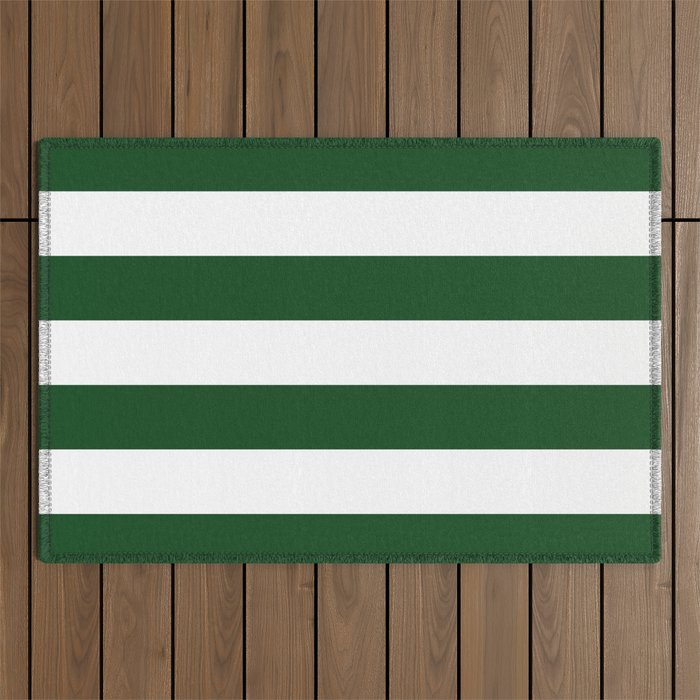The image depicts a large, square color photo featuring a medium brown wood tile floor as the background. The floor consists of vertical slats with small black gaps in between, running from the top to bottom, segmented by a single horizontal black line near the top. Central to the image is a tightly woven fabric, resembling a piece of canopy material or an outdoor tent cover, meticulously placed against the wood slats. This fabric displays alternating horizontal stripes in dark green and white, starting and ending with green, for a total of four green stripes and three white stripes. The fabric's edges are adorned with prominent white stitching, creating a slightly fringed outline around its perimeter. The wood planks with their light tone and dark grain emphasize the contrast with the structured symmetry of the striped fabric, highlighting its neatness and simplicity.